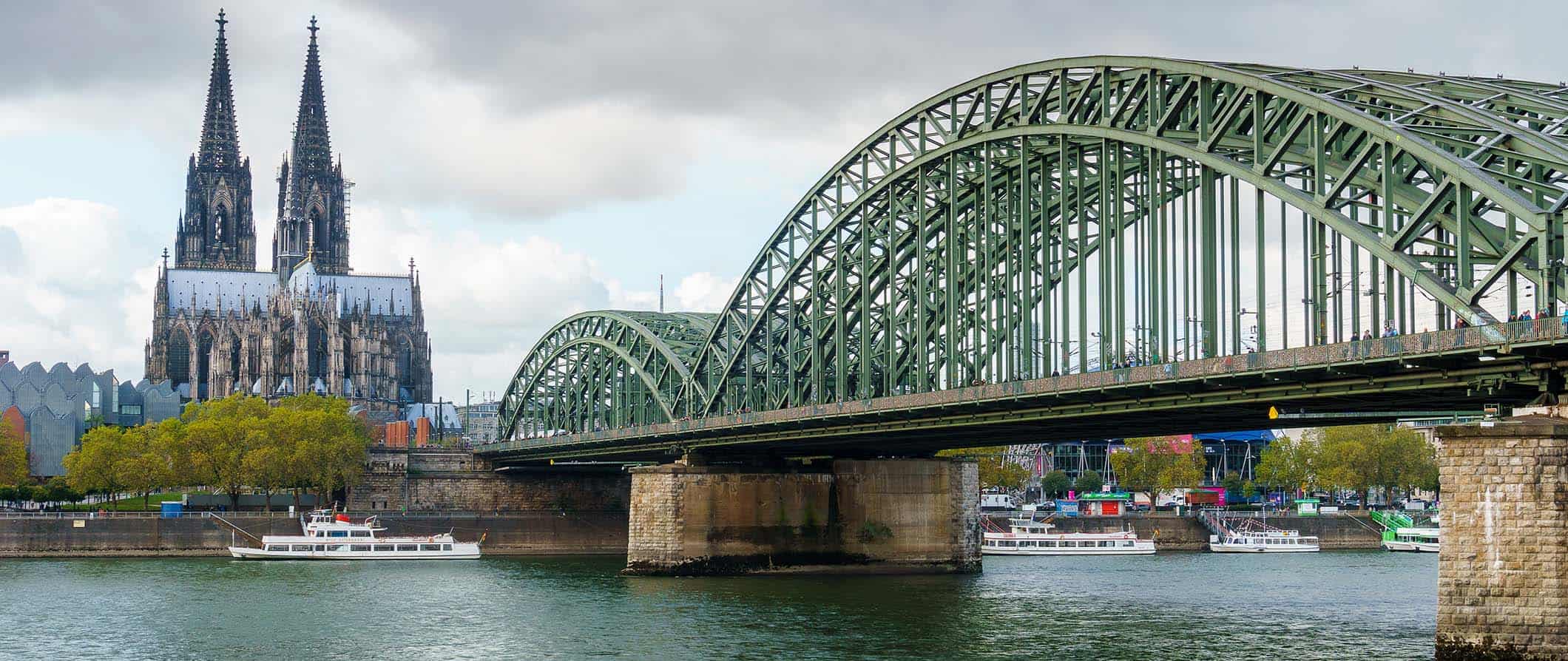The panorama image features a large, green bridge spanning a river, supported by metal girder arches that rise just slightly above the water. The bridge, characterized by its weathered sage or mint green color, includes two distinct arched sections and is held up by a brownish brick and concrete foundation, allowing ships to pass underneath. In the photograph's right foreground, some docked ferries are visible, while in the background to the left, a long white yacht appears to be navigating under the bridge. Dominating the left side of the scene is a formidable, twin-towered cathedral or castle, presumably from the 18th century. This imposing structure, with its tall spires capped by filaments, stands brownish with a white roof. The sky overhead is overcast, laden with gray clouds, though patches of blue sky peek through intermittently.